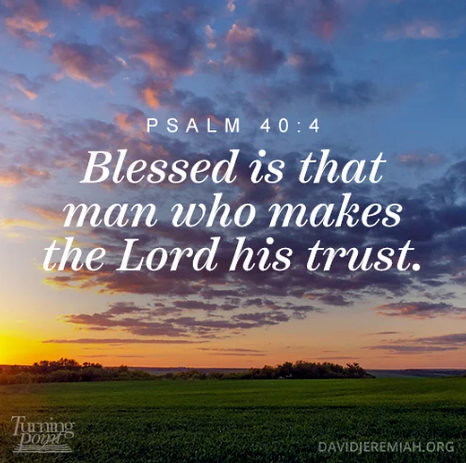The image is a small rectangular photograph, approximately four inches high and three inches wide, capturing the serene beauty of an outdoor scene during either sunrise or sunset. Dominating the top three-quarters of the picture is a vast expanse of sky which transitions from deep blue at the top to vivid orange towards the bottom, filled with scattered clouds showing various hues from orangish-purple to dark gray. Below the sky lies a panoramic view of a green grassy field with distant trees and foliage, potentially offering a glimpse of the ocean at the horizon. Printed centrally in bold white text is a verse from Psalm 40:4, "Blessed is that man who makes the Lord his trust." In translucent white print, the lower left-hand corner reads "Turning Point," while the lower right-hand corner features the website "DavidJeremiah.org." This atmospheric image conveys a sense of tranquility and faith, highlighting the connection between the natural world and spiritual reflection.